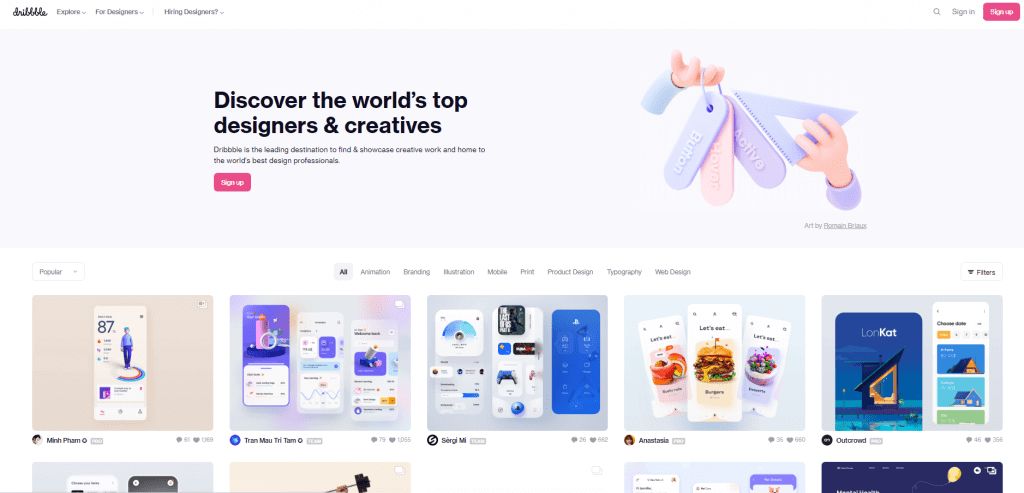The image depicts the homepage of a website titled "Dribbble," prominently displayed at the top. The navigation bar features buttons labeled "Explore," "For Developers," and "Hiring Designers." Below the header, a bold tagline reads, "Discover the world's top designers and creatives," setting the tone for the platform. Dribbble is described as a leading destination for finding and showcasing creative work, boasting a community of the world's best design professionals. A "Sign Up" button is also visible, inviting new users to join.

To the right, there's an illustration of hands holding name tags associated with design. Scrolling down, the page highlights a section labeled "Popular," showcasing a variety of visually appealing designs, which appear to be home screen mockups or similar creative assets. Each design has ratings and download numbers, though the specifics are somewhat hard to read.

A category bar is present, featuring sections such as "All," "Animation," "Branding," "Mobile," "Print," "Product Design," "Typography," and "Web Design." These categories organize the showcased designs, which are noted for their clean, professional, and well-executed nature, reflecting the site's credibility as a resource for high-quality design assets.